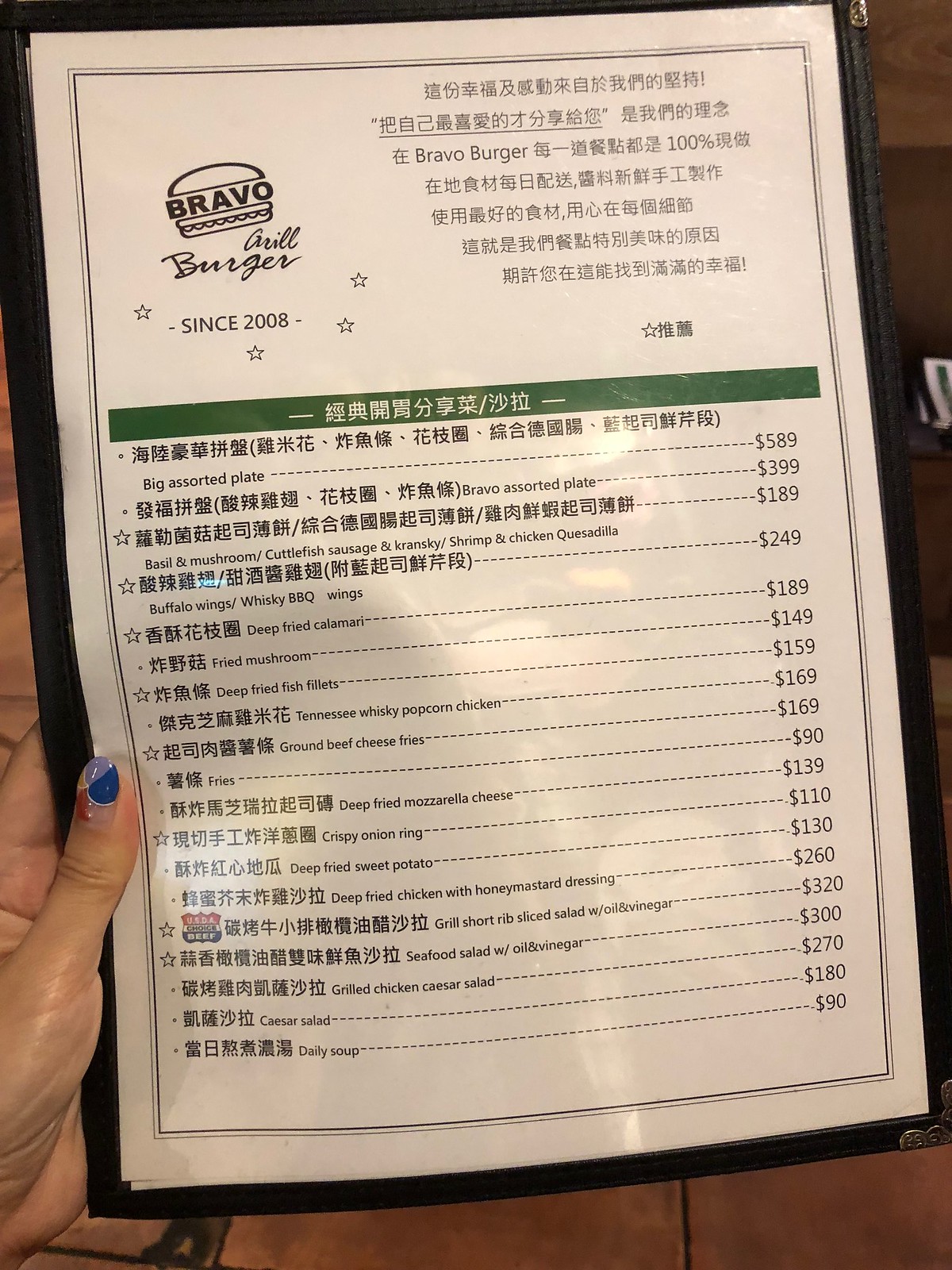In this image, a woman with chipped blue nail polish is holding a menu from Bravo Grill Burger, an establishment that claims to have been in business since 2008. The menu features predominantly Chinese text, written in black lettering against a white background, with a prominent green bar at the top. The menu items are curiously priced in what appear to be American dollar amounts, though the prices are unusually high, such as $589 and $399, adding a layer of confusion. The scene suggests that the menu is being held over a wooden surface, reminiscent of a picnic table. The juxtaposition of the English restaurant name and the Chinese menu text, along with the odd pricing, creates a puzzling visual composition.